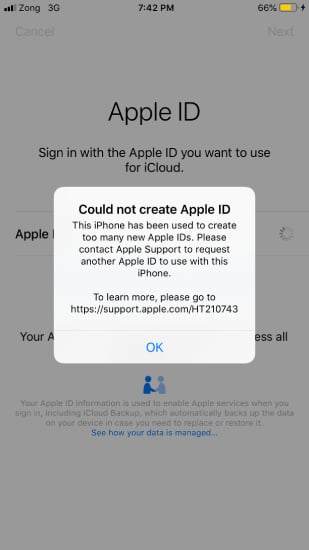The screenshot displays an Apple iPhone's screen at 7:42 p.m., connected to the Zong 3G network with a 66% battery life remaining, indicated by a gold-highlighted battery icon in the top-right corner. The background of the page is dark gray, and at the top, in all capital letters, it reads "Apple ID." The message instructs the user to sign in with an Apple ID to use iCloud. Below this, a white notification box states, "Could not create Apple ID. This phone has been used to create too many new Apple IDs. Please contact Apple Support to request another Apple ID to use with this iPhone. To learn more, please go to https://support.apple.com." At the bottom of the message, there's a clickable "OK" button. In the background, partially visible, is the word "Apple" accompanied by an image of two people shaking hands, one in blue and the other in lighter blue, with a prompt that says, "See how your data is managed."